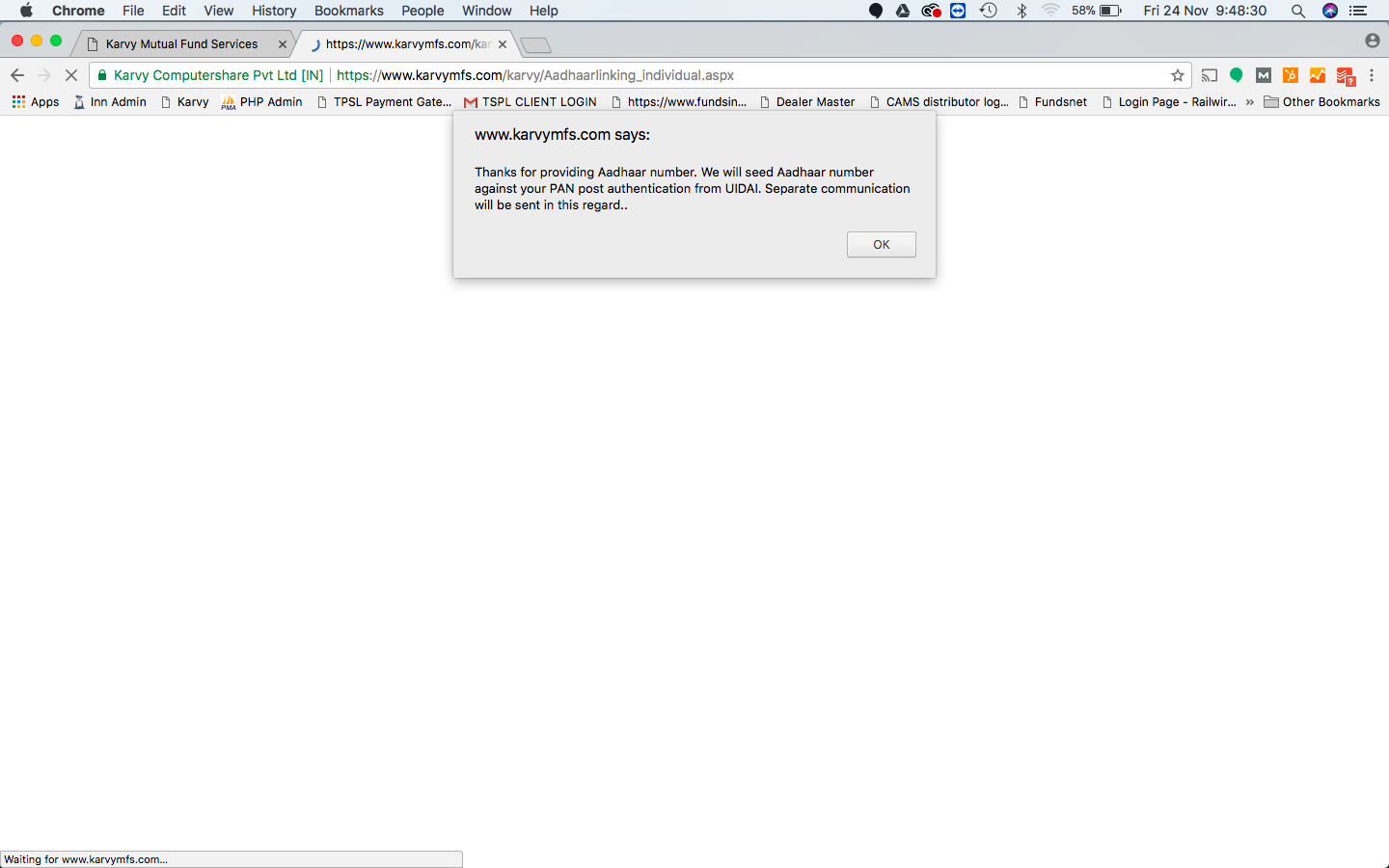The screen displays a browser window with the following details:

- The top menu bar includes options for Chrome, File, Edit, View, History, Background, People, Windows, Speech, and Google Drive.
- A red circle icon indicates a rotating element.
- The Wi-Fi status shows it is not connected.
- Battery is at 58%.
- The date and time are displayed as Friday, 24th November, 9:48:30.
- Window control buttons (red, yellow, green) are visible.
- The URL in the address bar is "https://www.carveymfs.com."
- The page belongs to Carvey Mutual Fund Services, associated with "Carvey Computer Share Private Limited."
- Additional links and tools listed include:
  - Carvey Add
  - Hire
  - Linking
  - Underscore Endorser.aspx
  - Apps
  - Admin
  - Carvey PHP Admin
  - TPSL Payment Gate
  - TSPL Client Login (https://www.funds.dealermaster.com)
  - Cams Distributor Log
  - Funds Net Login Page
  - Dash Robo

A pop-up message from "www.carveymfs.com" reads: "Thanks for providing our number. We will see that our number against your PIN, postal disclosure from you, IDEI, etc. Communication will be sent in this regard." The pop-up appears to be gray in color.